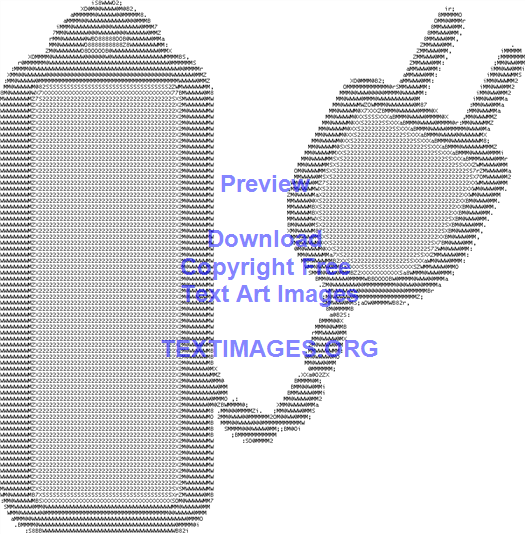The image showcases an intricately designed ASCII art representation of an electrical device, possibly a power strip or a water bottle with a power plug attached. This text art is created using a combination of letters and numbers, meticulously arranged to represent different shades and dimensions. The artwork stands against a white background, with darker text forming the outlines and lighter text filling the inner areas. Dominating the center of the image is a blue text watermark, centered and composed of multiple rows with one to three words each. The blue text reads: "preview, download, copyright-free text art images. textimages.org", indicating the source and nature of the artwork. This image emphasizes the creativity and complexity of text-based art and serves as a promotional piece for the website textimages.org, where such text images can be generated.